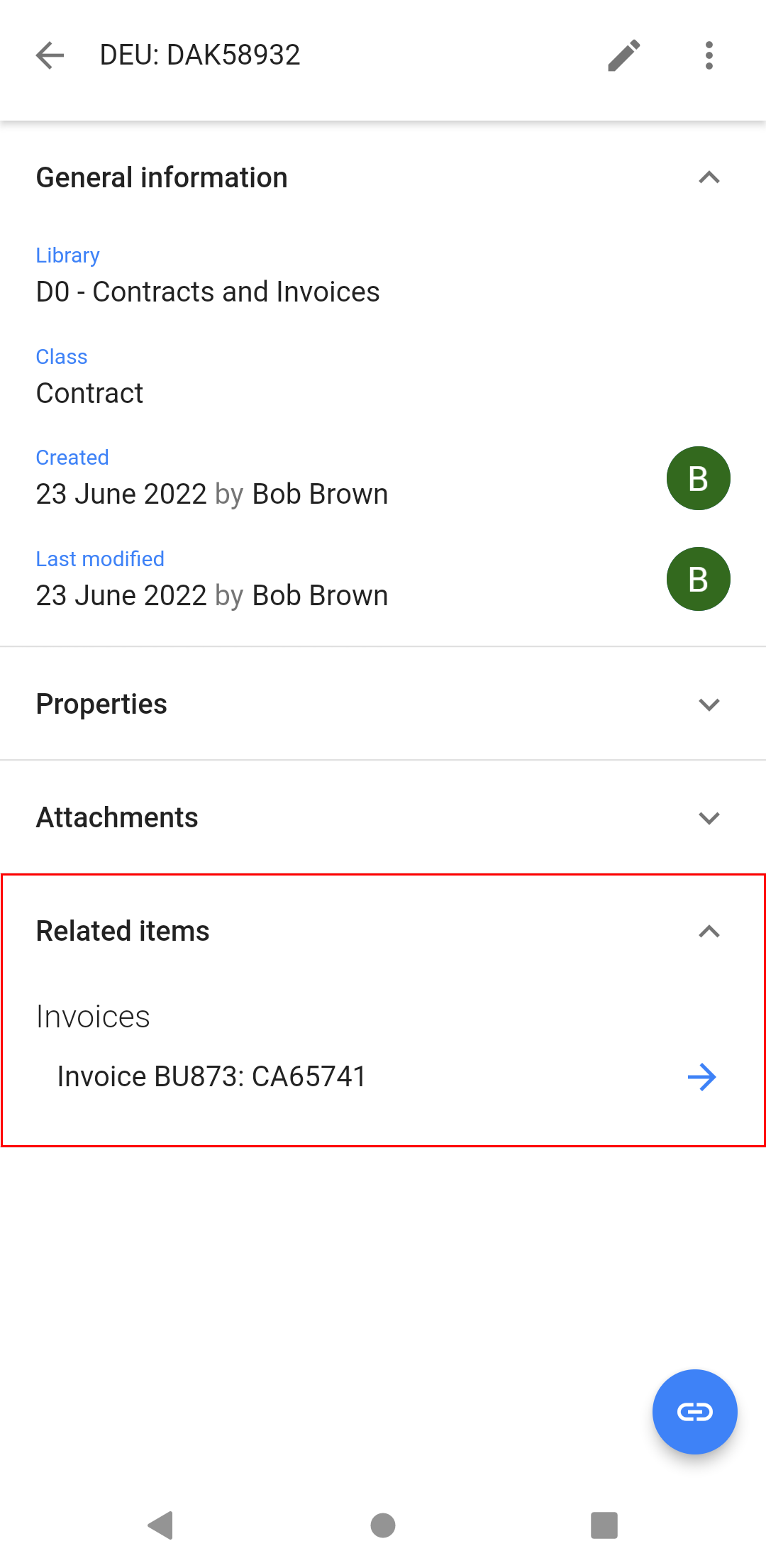This image displays a section from a phone screen with a white background. The top portion contains the header "General Information," followed by a title in blue reading "Library." Directly underneath, it states "DO-contracts and invoices" in black text. Below this section, there's another blue text marked "Class," with the word "Contract" written in black.

Further down, the document shows the creation information: "Created" is in black, succeeded by a blue text stating "June 23rd, 2022," and the name "Bobby Brown" in black. To the right of this creation info, there is a green circle with the letter "B" inside it. The "Last Modified" information follows next: "Last modified" in black, "23 June 2022" in blue, and "by Bob Brown" in black, accompanied again by a green circle with a B on the right side.

Below this, the words "Properties" and "Attachments" are listed in black text. Lastly, there is a prominent red box labeled "Related Items," which includes a subsection for invoices. Underneath the "Invoices" header, the specific invoice number is "invoice BU873CA65741," which is accompanied by a blue arrow pointing to the right.